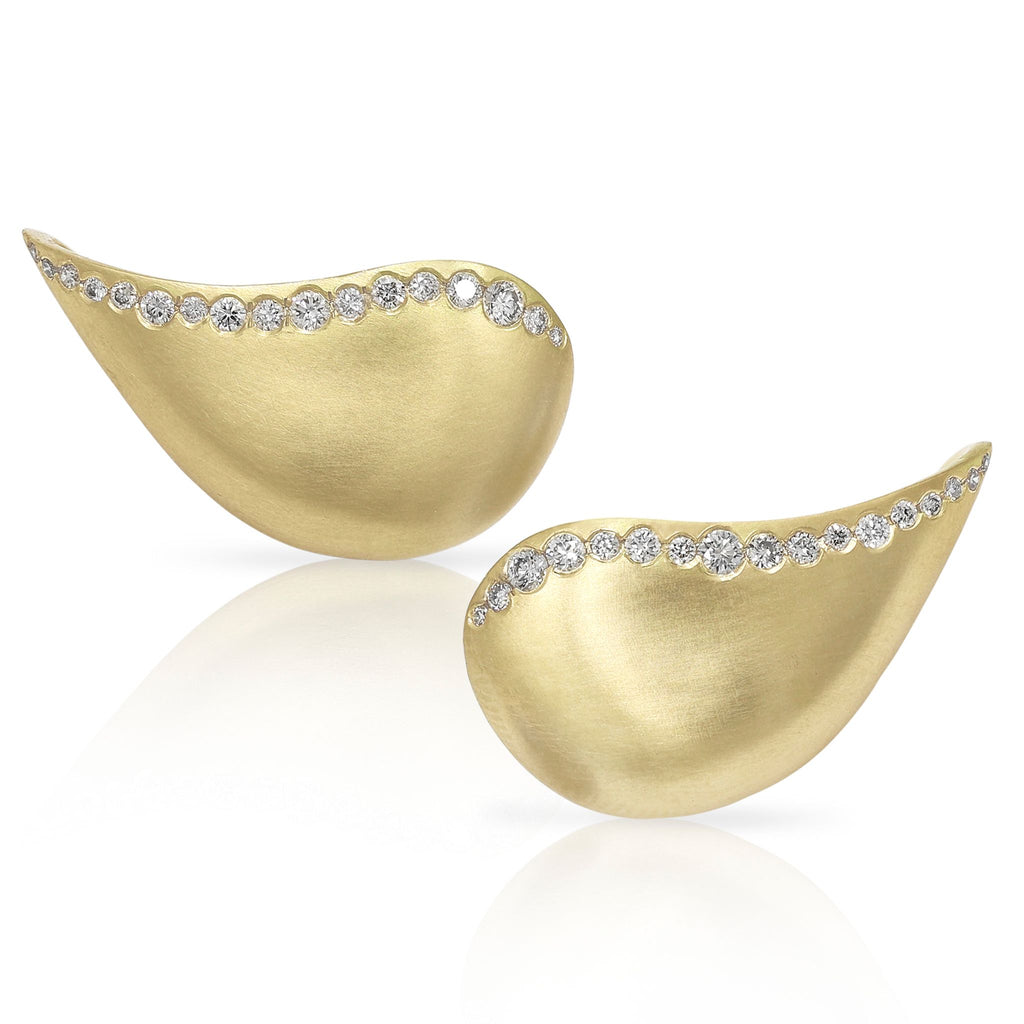The image showcases a pair of intricately designed teardrop-shaped ornamental pieces that exude an air of luxury and sophistication. These golden items, possibly earrings, are displayed against a white background, creating a shimmery reflection beneath them. The polished surfaces are highlighted with a rich brushed texture that enhances their gleaming appearance. Along the top edge of each teardrop-shaped piece, a line of various-sized diamonds is meticulously encrusted, starting from the pointed tip and slightly increasing in size toward the center and end. The diamonds’ brilliance complements the golden hue, making these items stand out. Their reflective surface casts subtle shadows on the ground, contributing to an overall impression that these are high-quality, likely gold, items elegantly presented, potentially for a luxury store's catalog.